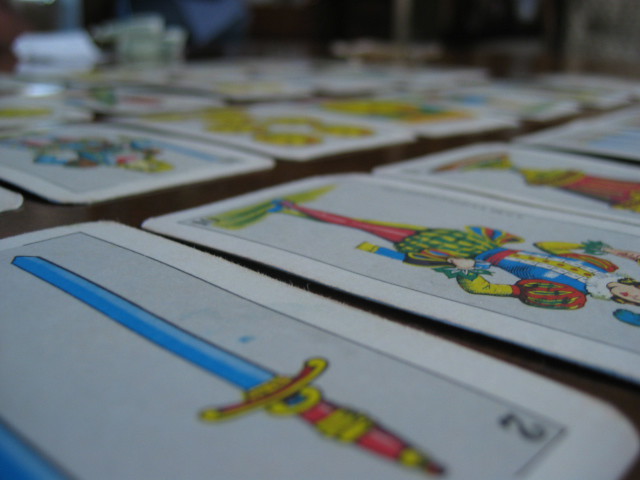This photograph captures a set of tarot cards laid out on a table. The background is blurry, revealing the end of the table where a person in a blue garment is seated. At the edge of the table, there appears to be some folded money or a white object, possibly a book, adding to the casual, everyday setting.

Focusing on the cards, each has a distinctive white border framing a gray center. The card closest to the viewer displays the number "2" in black in the corner and prominently features a sword. The sword has a yellow, gold-like hilt adorned with red stripes and some blue accents, while the blade itself is a periwinkle blue with a matching dot in the gray area of the card.

Next to this card is another, featuring an elaborately dressed figure, who appears to be a prince or a jester. This character wears a periwinkle blue top with a white frilly collar and billowy sleeves striped in red and green. Their attire includes a yellow section extending from the upper arms to the wrists and a short, poofy skirt in green and yellow, ending above the knees. Completing the outfit are vibrant red tights.